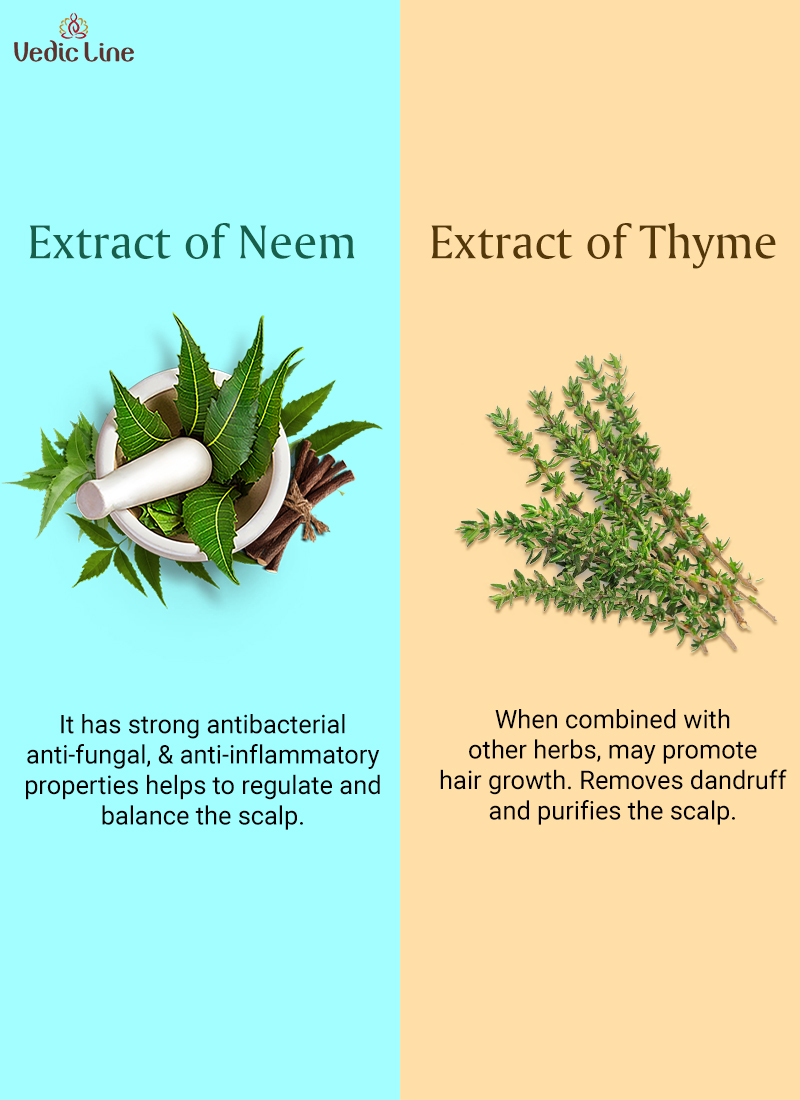This advertisement poster for Vedic Line features a detailed layout that is divided vertically into two halves: the left side showcases the "Extract of Neem" while the right side displays the "Extract of Thyme." The top left corner holds the Vedic Line logo. The left portion of the image has a teal background with the headline "Extract of Neem," accompanied by a photograph of green neem leaves placed in a white mortar with a pestle lying on top. The text at the bottom highlights the neem extract’s properties, stating it is strongly antibacterial, antifungal, and anti-inflammatory, helping to regulate and balance the scalp. The right half has a light brown background with the title "Extract of Thyme," and features several sprigs of thyme at its center. The text below explains that when combined with other herbs, thyme may promote hair growth, remove dandruff, and purify the scalp. This detailed and visually segmented design effectively communicates the benefits of neem and thyme extracts for hair care.